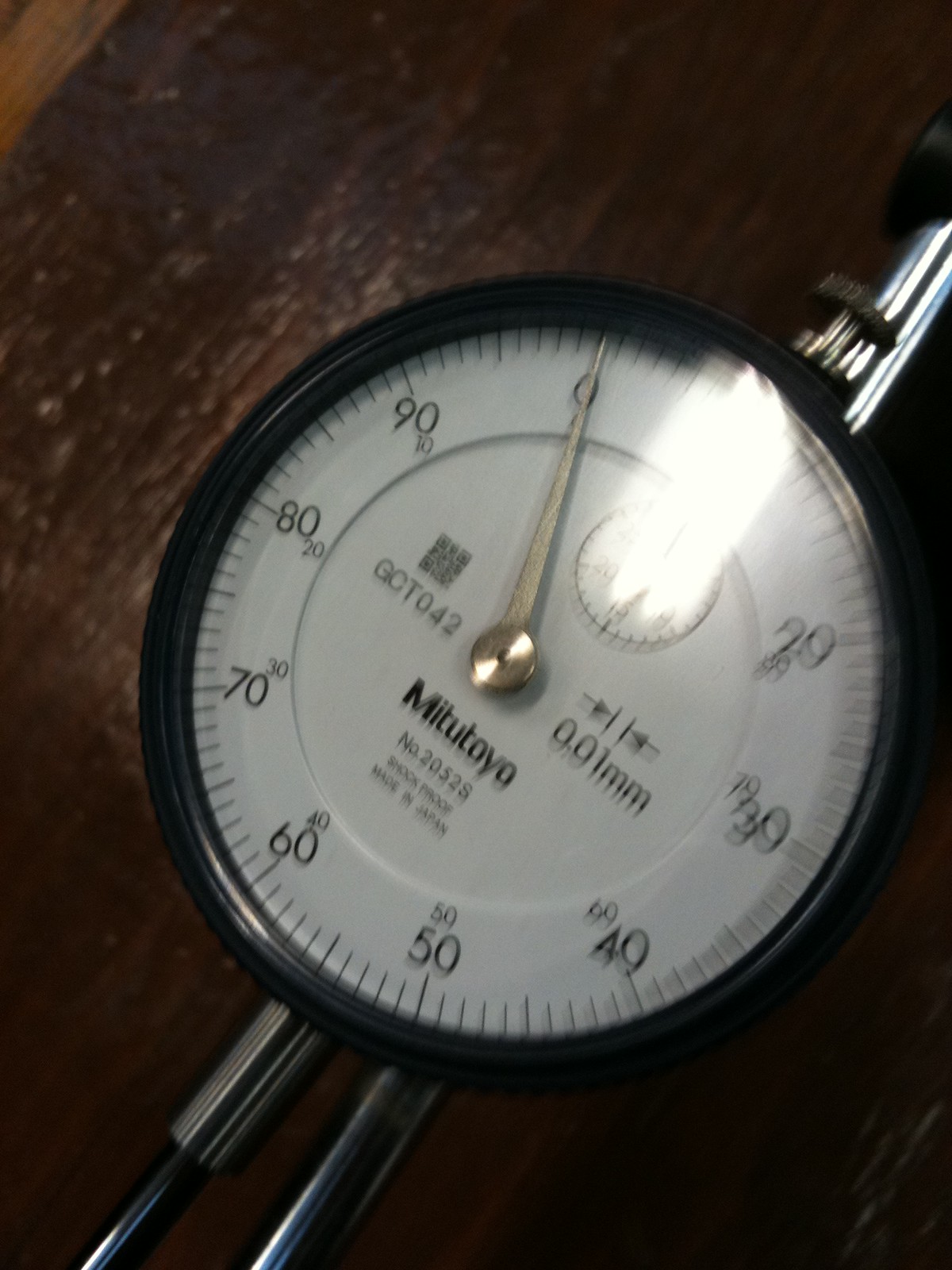This close-up image showcases a precision gauge, likely a dial indicator, resting on a rough-textured, medium-brown wooden surface. The pronounced wood grain and divots are particularly visible on the left side, highlighted by the bright overhead light that illuminates the top of the gauge.

The gauge itself is outlined in black and marked incrementally from 0 to 90 in units of 10, with smaller divisions indicating single units. A silver hand points precisely to the zero marker, anchored by a central silver pivot. The dial face bears the brand name "Mitutoyo," followed by the model number "2052S" below it.

On the left side of the dial, a small QR code is visible with the text "GC2042" adjacent to it. On the right side, the precision measurement "0.01 millimeters" is inscribed beneath two inward-pointing arrows bracketing a pair of vertical parallel lines.

The gauge is connected to an assembly of silver pipes, one extending from the top and another from the bottom, indicating its integration within a larger mechanical system.